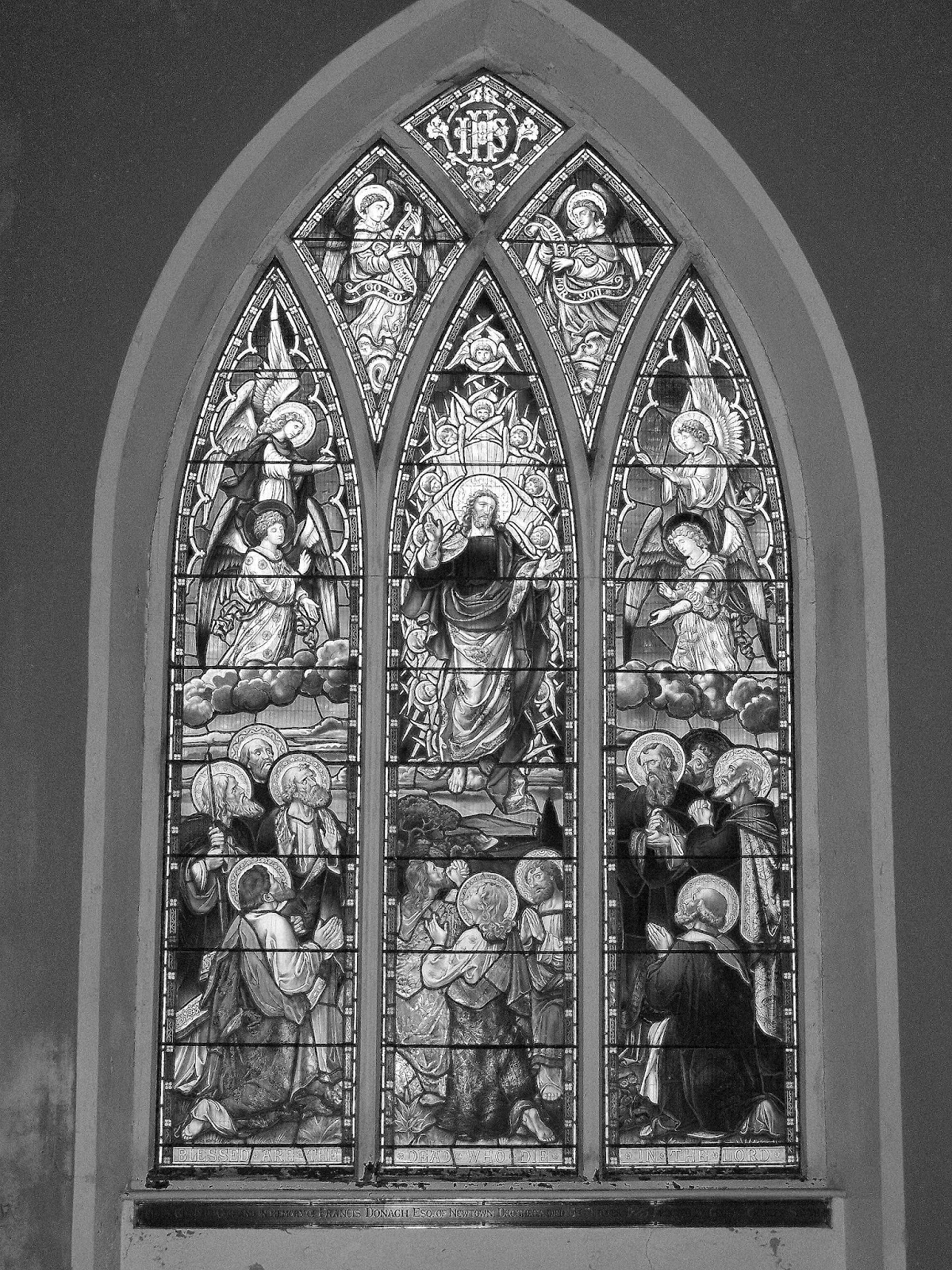This black and white photograph captures an intricate stained glass window in a church, showcasing an elaborate religious scene. At the center is a radiant Jesus with a halo around his head, his arms wide open, surrounded by numerous small angelic heads. Flanking Jesus are four angels, two on each side, adorned in long, flowing robes and some with halos. Positioned at the top corners of the window are two angels playing harps or similar instruments. 

Below Jesus, twelve men with halos, possibly the disciples or saints, are depicted. They are all gazing upward towards Jesus, with three of them on their knees in prayer, hands clasped. The bottom of the scene features more kneeling figures, enhancing the reverence and sanctity of the composition. Above it all, at the apex of the arch, there's a round circle bearing the inscription "IHS," possibly a Christogram.

This window, although captured in monochrome, conveys a complex and striking narrative adorned with detailed figures, halos, and flowing garments, reflecting the profound artistry typically seen in stained glass masterpieces.